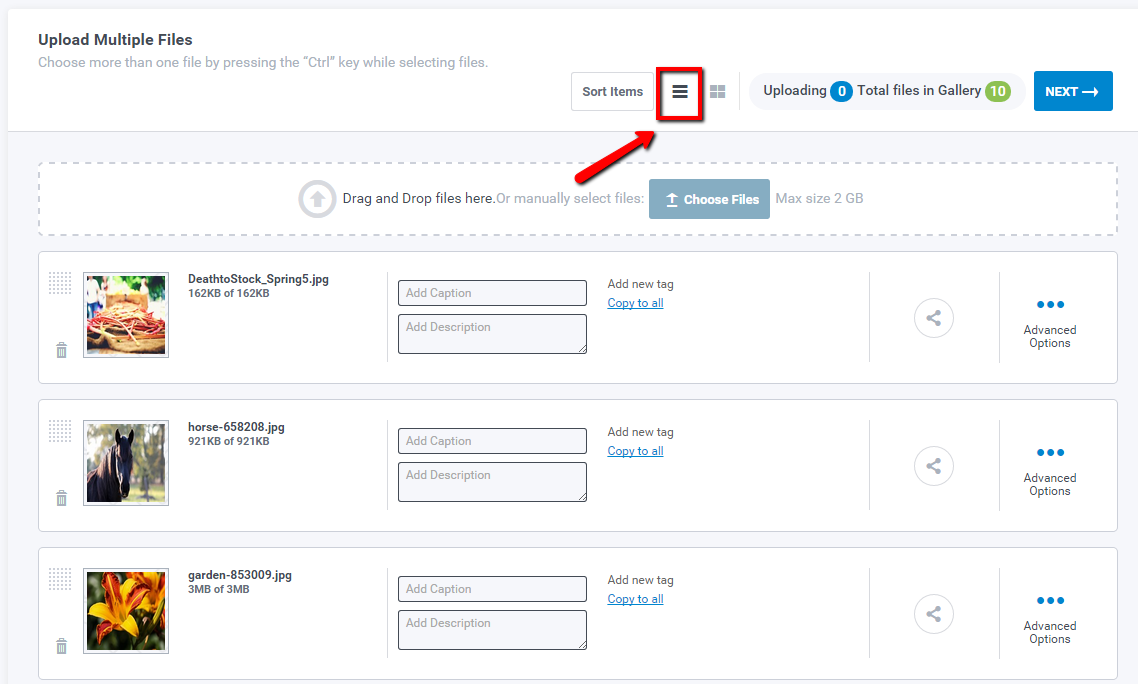This image showcases a file upload interface on a website with a light gray background. At the top, a white banner features prominently with the header "Upload Multiple Files" in black text, with the letters U, M, and F capitalized. Directly underneath, it provides instructions in smaller text: "Choose more than one file by pressing the 'Control' key while selecting files," with "Control" capitalized and in quotations.

Moving to the right, there is a square button labeled "Sort Items." Adjacent to this are two icon buttons: one is a white square with three black lines enclosed by a red border, and the other is a composite of four small squares forming one larger square. An arrow points upward to the icon encased in the red border.

Below this area, another interactive element shows a progress tab indicating "Uploading 0 Total Files" with "0" on a blue background and "10" on a green background. To the right of this progress indicator, there is a blue tab labeled "Next" with white text.

Further down, a second white banner bounds a designated upload area outlined by a dotted line. This area prompts the user with the text "Drag and drop files here or manually select files." Inside this area, there is a blue-gray button with white text that reads "Choose Files." Below this button, it specifies a maximum file size of 2 GB.

At the bottom of the image, three uploaded file thumbnails are displayed with their respective filenames:

1. "death_to_stock_spring5.JPG"
2. "horse-658208.JPG"
3. "garden-853009.JPG"

Each filename indicates the type of content (a spring image, a horse, and a garden flower) alongside its format and file number identifier.